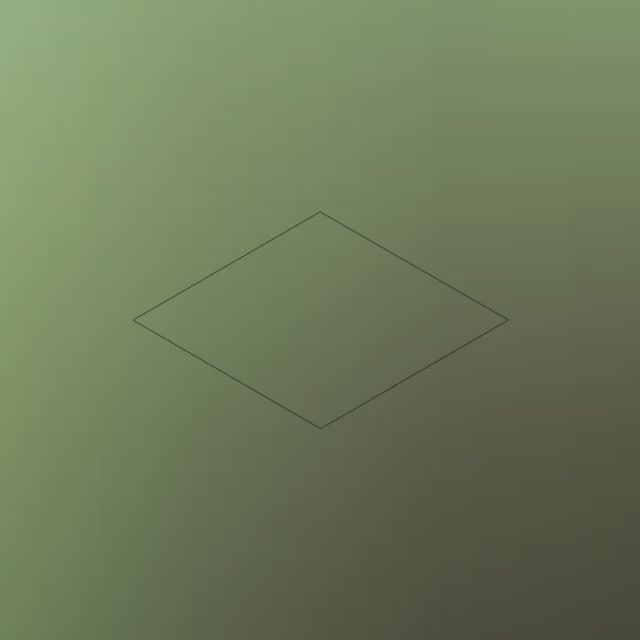The image depicts a piece of paper with a gradient background, transitioning from a light olive color in the upper left to a darker olive in the bottom right. The surface has no visible blemishes and appears smooth, but it features some distortion or artifacting that makes it look slightly blurry. Dominating the center of the paper is an outline of a shape that resembles both a square and a diamond, drawn with a thin black line. The shape, which has no fill or borders, can appear as either a square or a diamond depending on the angle from which it is viewed. The entire image maintains a very minimalist aesthetic, with the outline being the only notable detail against the gradient background.